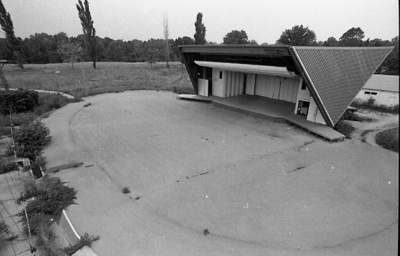The black and white photograph depicts a small, uniquely triangular-shaped building, reminiscent of a bus stop or shelter. The structure features sides that resemble inverted triangles with pointed bases, supporting a roof and possibly housing lockers or similar rectangular elements inside. This shelter is positioned in the upper right part of the image. It stands on a roughly circular or ovular driveway, possibly intended for vehicles to maneuver around and exit from the same lane. 

Surrounding the building, there is a blend of nature and concrete; a field of grass extends to one side, punctuated by a few evenly spaced slender trees, leading to a denser forested area in the background. The driveway itself shows signs of wear, with grass growing through its cracks. A road is also visible adjacent to this scene. The overall ambiance is vintage, enhanced by the black and white tones of the photograph.